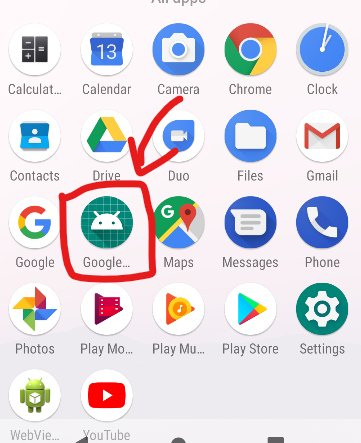In this cell phone screenshot, the background is entirely white, providing a clean and clear contrast for the icons displayed. The top portion of the image appears to have been cut off, but a glimmer of text suggests it could be labeled "My Apps." 

The top row of circular app icons includes a calculator app, a calendar app, a camera app, a Chrome app, and a clock app. These circular icons represent a distinctive design choice, differing from the more traditional square icon shapes on some other phones.

The second row features a contacts app, a Drive app, a Duo app, a files app, and a Gmail app. Below this, the middle section displays a Google app, a partially visible application labeled "Google..." with an ellipsis, a Google Maps app, a messaging app, and a phone app.

As we move further down, the third section showcases icons for a Photos app, a Play Movies app, a Play Music app, a Play Store app, and the settings app. Adjacent to these, there is a web browser app labeled 'V' and a YouTube app.

Additionally, someone has drawn a haphazard square around the "Google..." application and added an arrow pointing towards it, drawing attention to this specific icon.